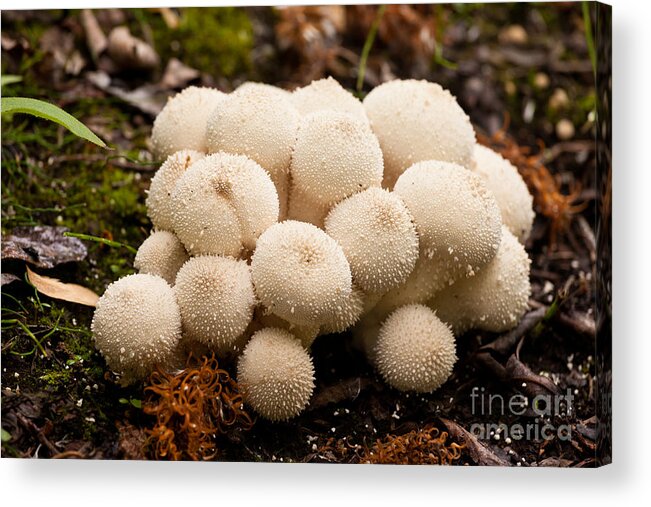This is a detailed, up-close photo printed onto a block, designed for hanging as artwork. The image focuses on a large cluster of white and beige fungal growths, resembling fuzzy balls with small spikes or particles sprouting from them. Approximately 20 mushroom-like formations of various sizes are tightly clumped together, situated on a damp, leafy ground that appears recently moistened by rain. The earthy setting features green leaves, brown dirt, weeds, grass, and wood fragments. In the lower right-hand corner, the text "Fine Art America" is subtly inscribed.